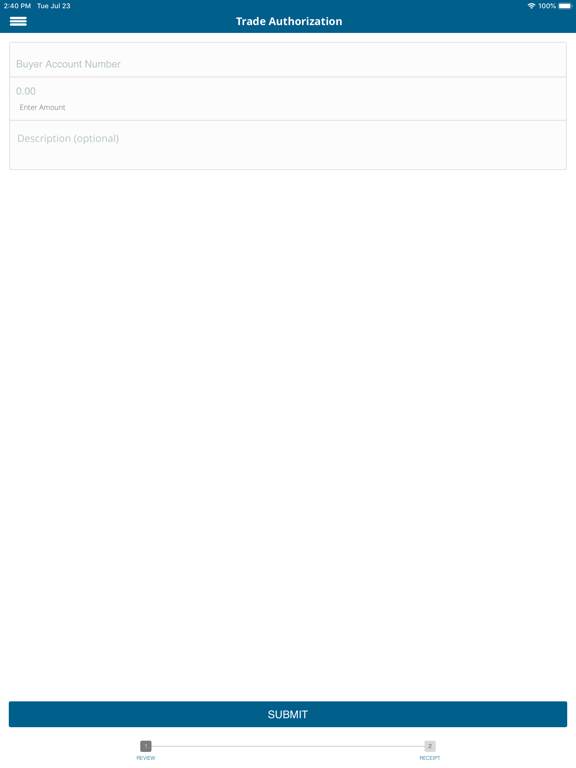The image depicts a stock trading website interface where financial transactions are conducted. In the top left corner, there is a blue rectangle displaying the current time, "2:40 p.m.", and the date, "Tuesday, July 23rd." The top right corner features a Wi-Fi symbol indicating a full 100% signal strength, alongside a battery icon signifying full charge.

Below this, towards the left, are three horizontal lines, possibly representing a menu. Centered on the screen is a prominent blue rectangle with white text reading "Trade Authorization."

The interface contains three main input fields. The first field, labeled "Buyer Account Number," is a text input area. The second field, "Enter Amount," accepts currency or numerical values. The third field, labeled "Description," is optional and indicated as such next to the label. These fields are designed in shades of gray against a white background.

At the bottom of the screen is a long blue submit button, consistent with the color of the top bar, featuring the word "Submit" in white text. Directly below the submit button are two step indicators: "1. Review" and "2. Receipt," connected by a line. The "Review" step is currently highlighted, suggesting that upon submission, the process will move to the "Receipt" step where the transaction details can be reviewed.

Overall, the interface is clean and functional, guiding the user through a step-by-step process for authorizing a trade.